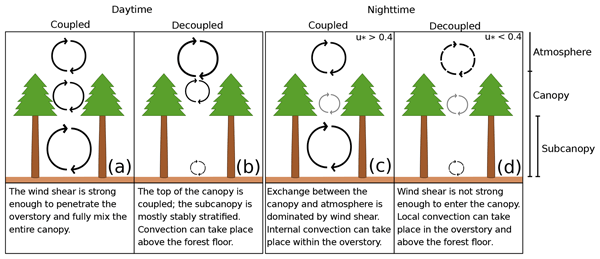The image is a detailed scientific diagram divided into four sections, each illustrating different conditions of wind interaction with a forest canopy during daytime and nighttime. The sections are labeled A (daytime, coupled), B (daytime, decoupled), C (nighttime, coupled), and D (nighttime, decoupled). Each section features two computer-animated trees with green, fur-like canopies and brown trunks, resembling Christmas trees. The background includes three vertically aligned labels on the right side: atmosphere, canopy, and sub-canopy. 

Section A describes that wind shear is strong enough to penetrate the overstory and fully mix the entire canopy. Section B notes that the top of the canopy is coupled, while the sub-canopy remains mostly stably stratified, allowing convection above the forest floor. Section C indicates that an exchange between the canopy and atmosphere is dominated by wind shear, with internal convection occurring within the overstory. Section D states that wind shear is insufficient to penetrate the canopy, causing local convection to occur in the overstory and above the forest floor. Each section is accompanied by curved arrows symbolizing airflow patterns through the trees. The main colors in the image are green and brown, representing the trees and their trunks.